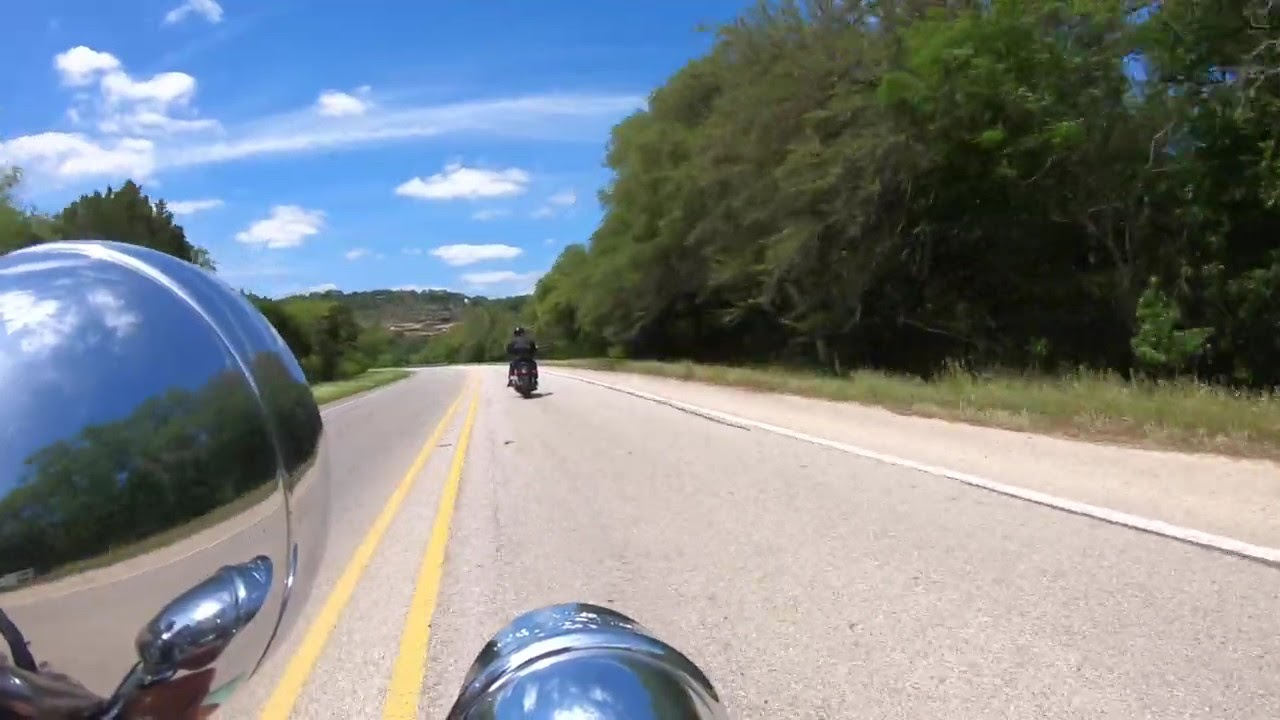In this close-up GoPro image taken from the perspective of a motorcyclist, we see a vivid scene unfolding on a single-lane highway surrounded by greenery. It's midday, with a few clouds dotting the blue sky. The image primarily captures the front lights and handle of the photographer's silver motorcycle at the bottom left of the frame. Ahead, a motorcyclist in a black jacket rides along the center of the road, slightly distanced but clearly visible. There is an absence of other vehicles or pedestrians, emphasizing the remote, serene surroundings with trees and grass lining the roadside. In the far distance, past the green hills, there appears to be a faint outline of a building or town. The scene is awash in natural colors: greens from the foliage, grays, and silvers of the bikes, the black of the motorcyclist's jacket, and the earthy tones of the landscape. Yellow lines divide the road, reinforcing the direction of travel and the sense of an open, uninhabited pathway ahead.